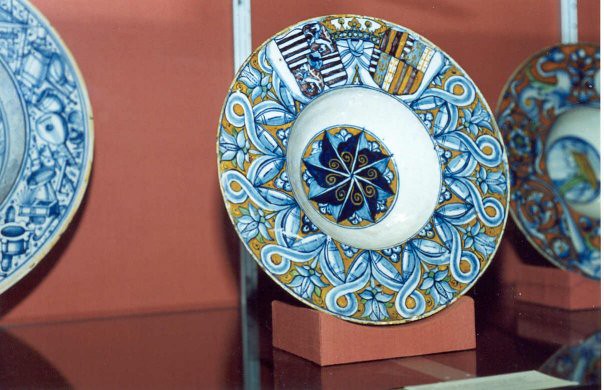This is a color photograph prominently featuring a decorative plate with intricate and vibrant designs, displayed in a display case that might be open. The plate stands upright on a terracotta-colored stand, against a matching terracotta background. The plate exhibits a busy design that includes blue, light blue, navy blue, powder blue, gold, and white colors. The outer rim features looping patterns in blue and gold, and the central part of the plate has a white background with a goldenrod circular area in the middle, depicting a prominent dark blue flower with gold swirls, resembling a pinwheel. To either side of the central plate, the photo captures partial views of two additional plates with similar Mexican-inspired designs in powder blue, white, and gold. The plates are all displayed on a black shelf, with no visible text, people, or location identifiers.